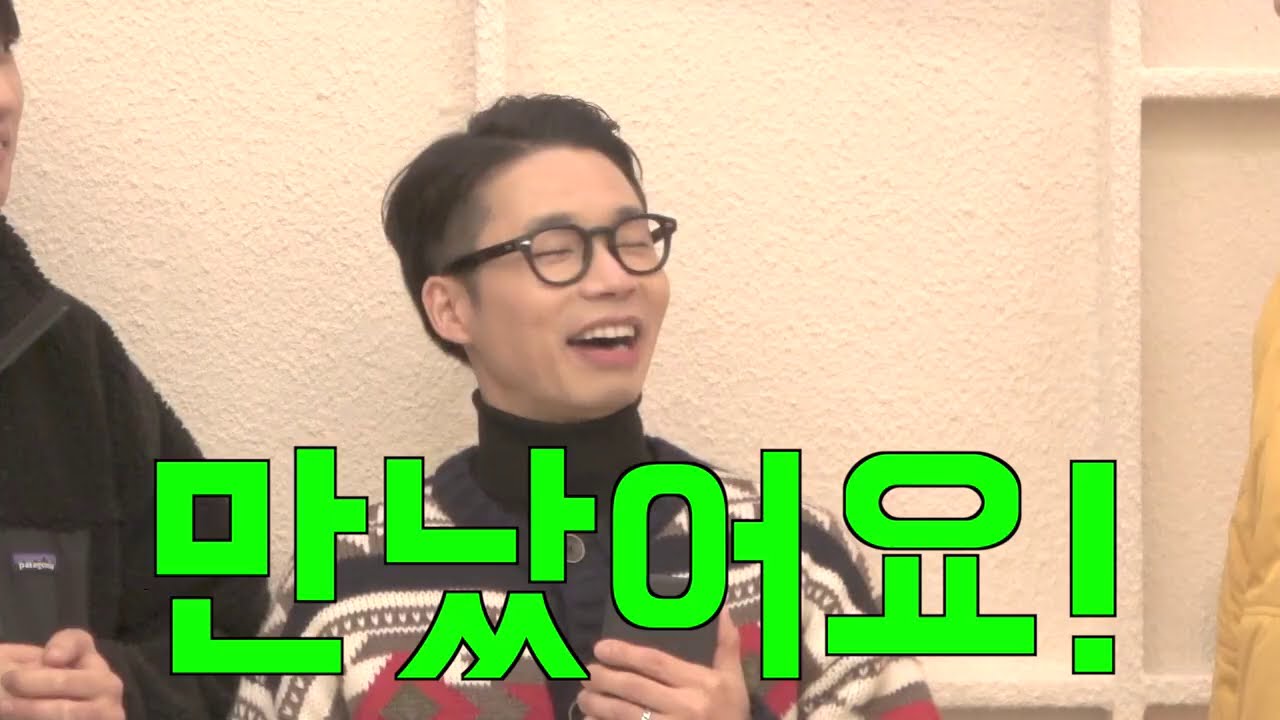In this photograph, an Asian man with short black hair and round black glasses stands against an off-white, textured wall. He is wearing a black turtleneck and a multicolored knit sweater with a pattern of black, white, gray, and red. The man's left hand is held up at chest level, holding a cell phone facing him. He is smiling broadly, his eyes squinted shut, and his head slightly tilted upwards as he looks to the right. 

Next to him on the left is a taller man, partly cut off at the edge of the photo, wearing a fuzzy, zip-up Patagonia jacket. Additionally, there is a hint of someone on the right side of the image, indicated by a small visible section of a yellow jacket. 

The image also includes bold, neon green text in an Asian language, possibly Korean, with a black outline around the characters, positioned at the bottom of the photo.